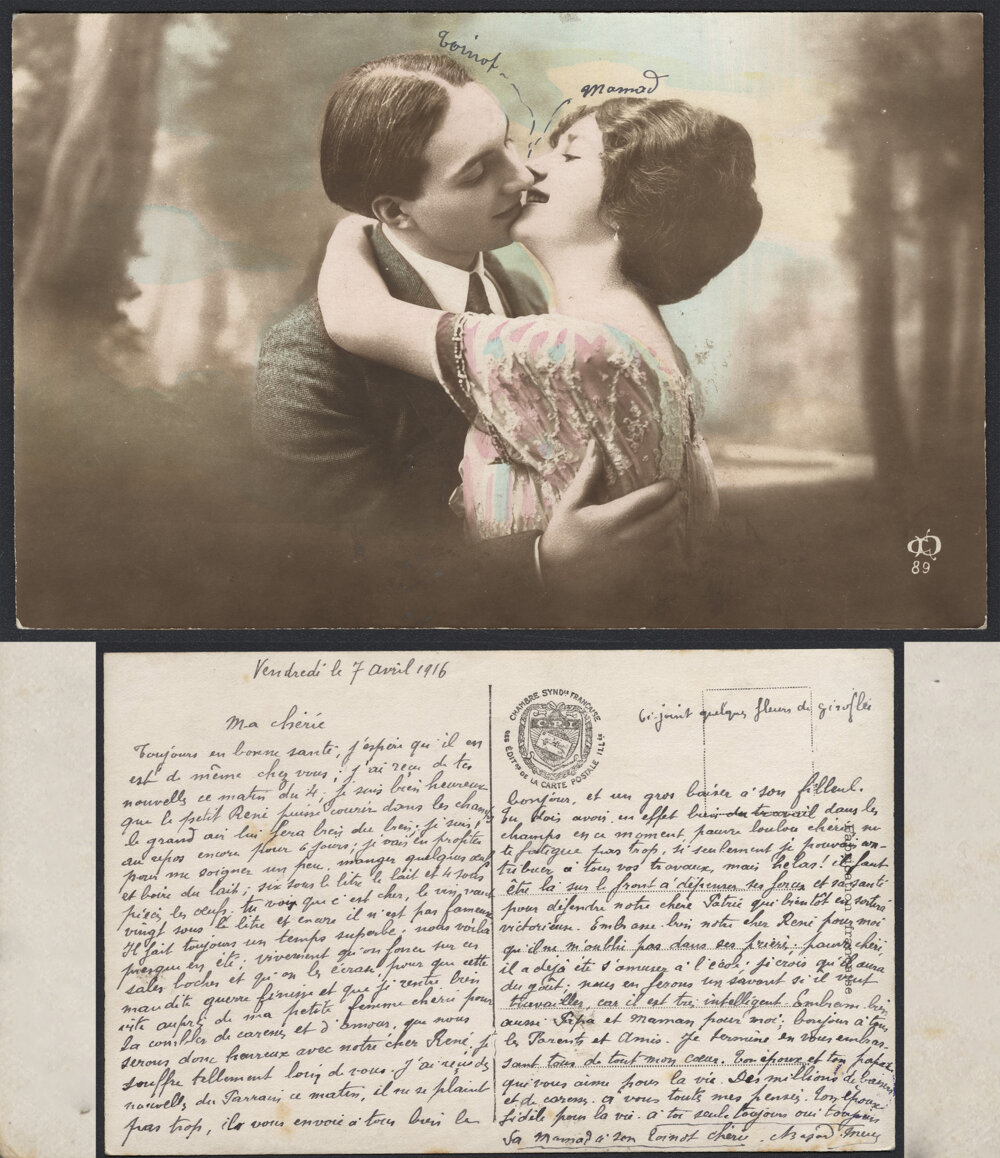The image portrays a black and white photograph at the top of a vintage postcard dated April 7, 1916. The photograph features a young couple deeply and passionately kissing, with the man sporting hair parted in the middle and the woman with short, wavy hair. The postcard is filled with handwritten notes in French, addressing "my dear" and wishing "always in good health." The writing covers much of the postcard in two columns and includes a stamp and a seal that reads "Chamber S-Y-N-D Francaise, Edite de la carte postale" with "CPI" visible as well. This appears to be an intimate love letter, preserving a moment of affection and care from over a century ago.